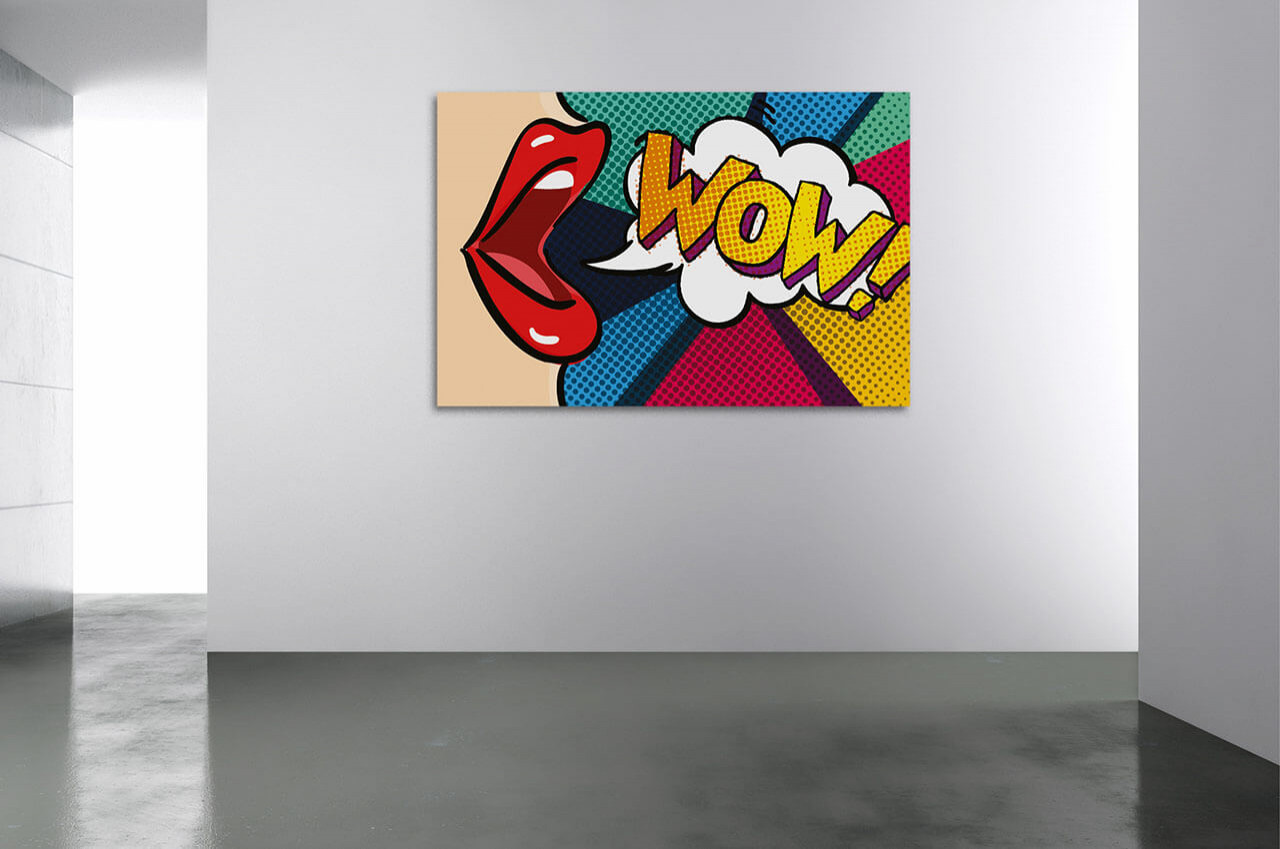The image is of a spacious room with white walls and a gray cement floor that has a shiny appearance. At the focal point is a striking pop art painting, reminiscent of Roy Lichtenstein's style, prominently displayed on the back wall. The painting features a cartoonish depiction of a woman's lips, rendered in bright red lipstick, her open mouth revealing her teeth and tongue. This section of the painting is surrounded by a pattern of dots in various colors, a hallmark of pop art. Emitting from her mouth is a white speech bubble with the yellow word "WOW!" outlined in black and accented with purple polka dots. The background of the painting showcases a vibrant pinwheel or sunburst pattern with segments in teal, blue, red, yellow, and black, further emphasizing the dynamic and colorful nature of this artwork. The overall scene exudes a modern and minimalist aesthetic, possibly indicative of a gallery or a contemporary home setting.